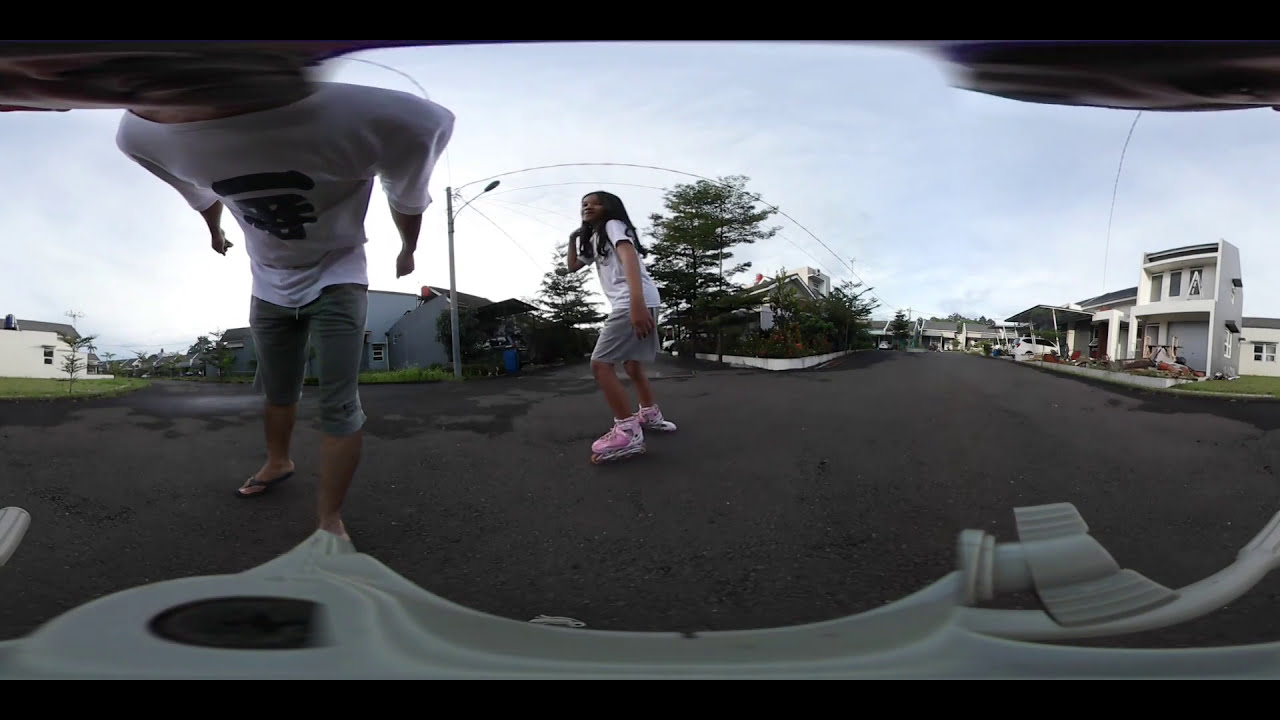The image depicts a distorted, wide-angle view through a windshield of a residential street during daytime. Dominating the center, a young girl with black hair cascading to her chest is seen wearing a white t-shirt, black shorts, and pink roller skates, gliding along the dark gray asphalt street. To her left, a person stands leaning forward, partly cropped out of the frame, wearing a white shirt with a black emblem divided into two parts, gray shorts just below the knees, and black sandals. The left side of the background reveals white-walled buildings with flat roofs, one featuring a carport sheltering a white car. Centered behind the figures, tall green trees rise against a backdrop of a slightly cloudy, light blue sky, adding depth and a sense of a peaceful neighborhood setting to the image.